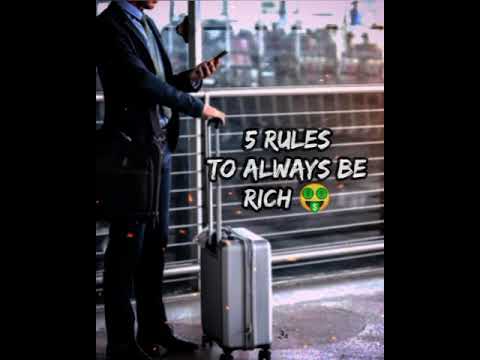In the image, a man is standing on the left side with his face out of frame. He’s wearing a dark blue blazer over a light blue button-down shirt, paired with blue jeans and black shoes. Over his right shoulder, he has a black messenger bag. With his left hand, he is looking down at his phone, and with his right hand, he is holding the handle of a small silver-gray carry-on suitcase with wheels. Behind him, a train station and the skyline of a city are visible. The text in the center-right of the image reads "Five rules to always be rich," accompanied by a smiley face emoji with dollar signs for eyes and a dollar sign as its tongue. The overall impression is that of a social media advertisement with a motivational quote.